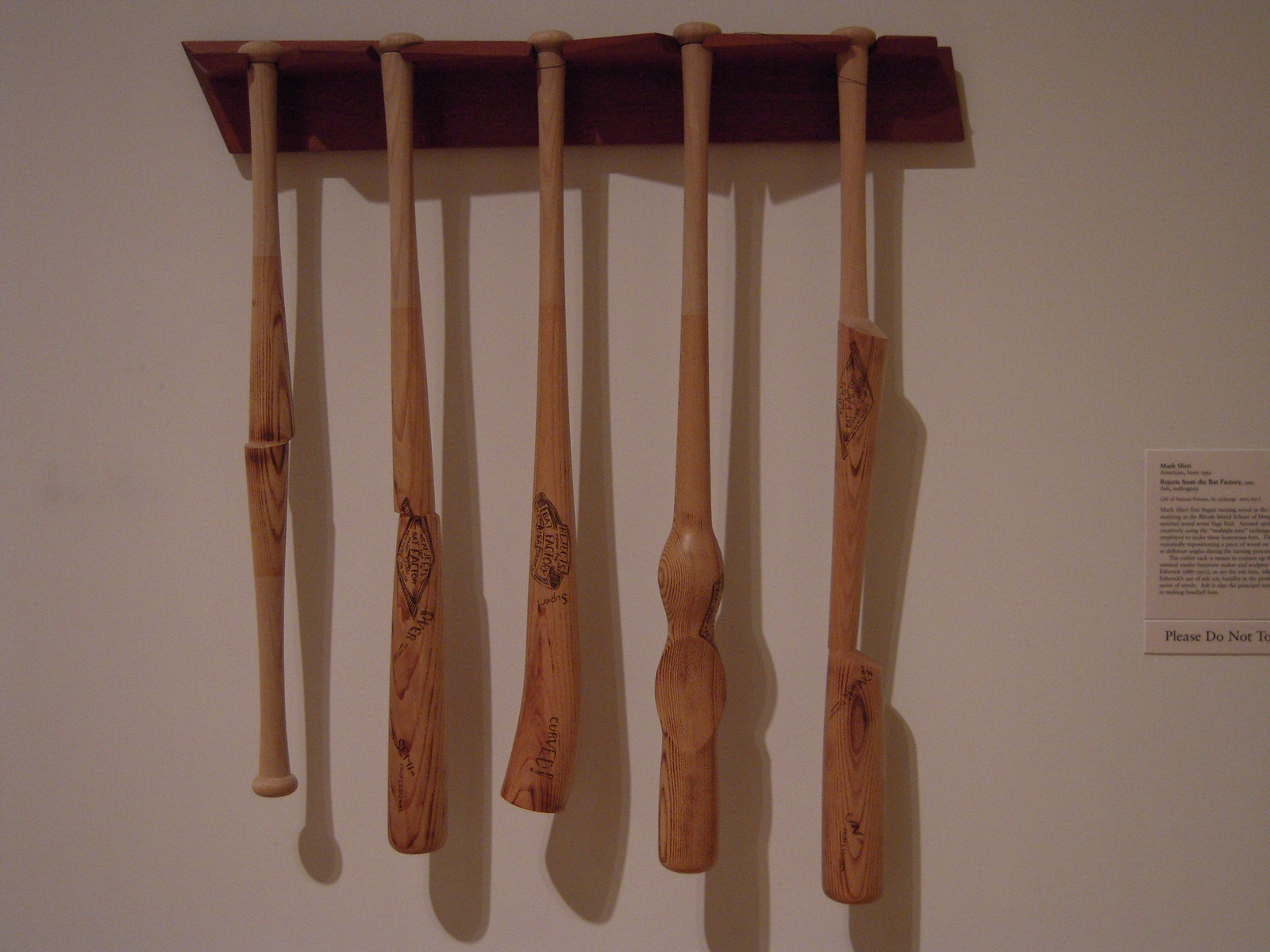The image captures a chestnut-brown wooden rack mounted on a white-gray wall, supporting five intricately carved wooden objects that, at first glance, resemble elongated baseball bats. Each piece exhibits a unique and elaborate design, distinct yet cohesive in their material and craft. 

From left to right, the first object resembles the end of a knitting needle and appears to be two shorter bat-like sections joined at the center, showcasing pronounced wood grain and subtle dark veins. The second item is more traditional in shape, widening as it extends down with a rich grain pattern and potentially engraved details. The central object starts as a conventional bat but transitions into a flatter, rounded end with intricate filigree carvings.

The fourth piece departs from traditional shapes, featuring an extended handle with two oval, bulbous protrusions along its length, adding a dynamic flair. Lastly, the rightmost object is the longest, initially akin to a baseball bat but transforming into a more abstract form with pronounced curves and a triangular section before tapering to a wider end. The underlying shelf has cutouts that securely hold each carved item.

Casting shadows on the wall, these objects collectively create an artistic display, accented by a nearby sign that reads, "Please do not touch," urging viewers to admire the craftsmanship without physical interaction.